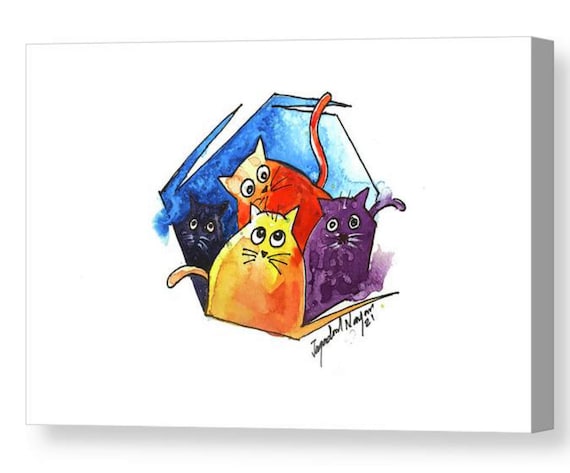This artwork is an illustration of a 3D canvas painting, giving the illusion of being raised off a wall with a shadow on the right side. The canvas features a white background in a landscape ratio, with a jagged, almost hexagonal, blue and white watercolor shape in the center, occupying about 30% of the canvas. Inside this geometric shape, four cats are depicted, each with large eyes and distinct colors. The cats' colors are black, red, deep purple, and yellow. Specifically, the black cat has white whiskers and yellow eyes, the red and yellow cat has white eyes with black pupils and a large orangey-red tail, the purple cat features a dual-tone of dark and light purple with white whiskers, and the yellow cat has black whiskers and white eyes. Below this geometric shape, the artist's signature is present, followed by the number 21, suggesting the creation year as 2021.